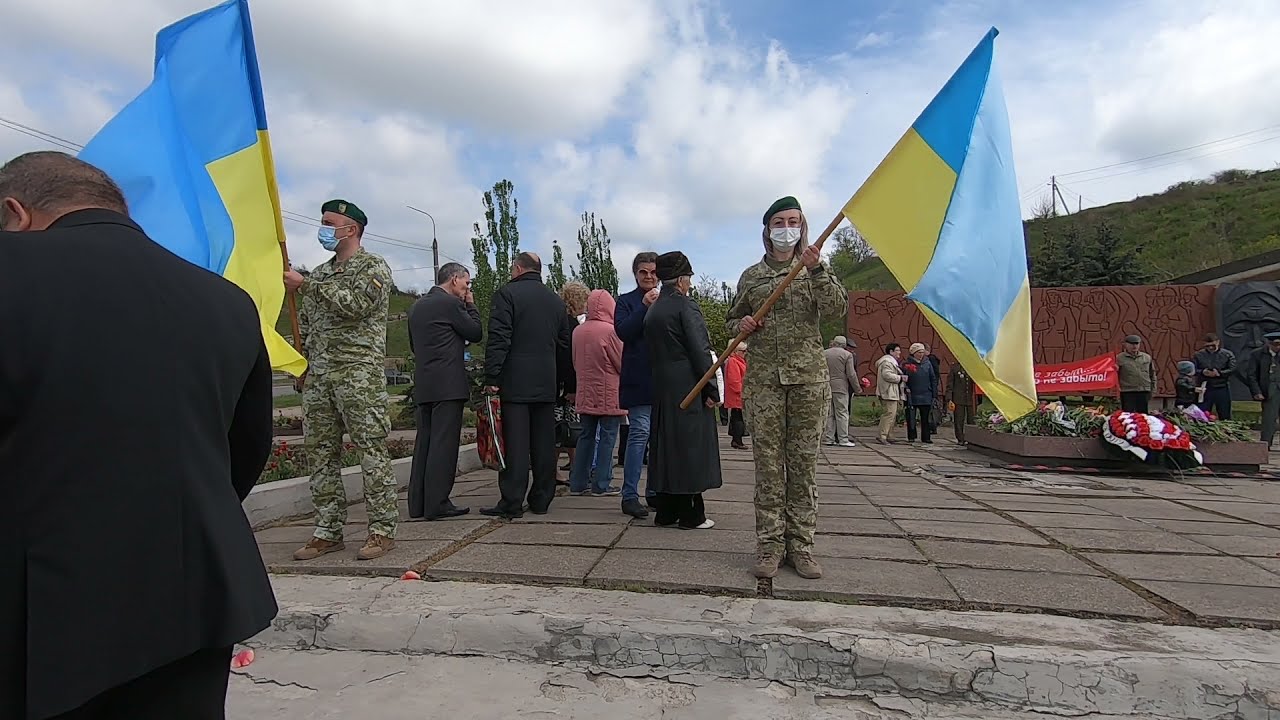In a horizontally aligned photo taken outdoors, a solemn gathering is evident during a memorial service. The sky is a light blue with patches of large gray and white clouds, suggesting a rather chilly day as indicated by everyone wearing jackets. Multiple individuals are present, many dressed in dark suits and long jackets, standing on a raised step. The focal point of the image showcases two soldiers, a man on the left and a woman on the right, both donning green camouflage uniforms, brown boots, and green berets with yellow emblems. These soldiers, who are also wearing face masks, are holding flagpoles with flags that are half blue on top and half yellow on the bottom, resembling the Ukrainian flag. To the left, a man in a black suit with short brown hair is seen facing away from the camera.

Behind the soldiers, a large floral arrangement of red and white flowers can be observed, indicating a flower laying ceremony. The background reveals a large green hill, and towards the right of the image, there is a memorial site surrounded by people who appear to be socializing yet partaking in the solemn event. The ground in front of the attendees is cracked and gray, enhancing the scene’s somber atmosphere. The image captures a poignant moment, likely a funeral procession or a memorial service for those who have perished in war, drawing a significant crowd of mourning individuals to honor the fallen.